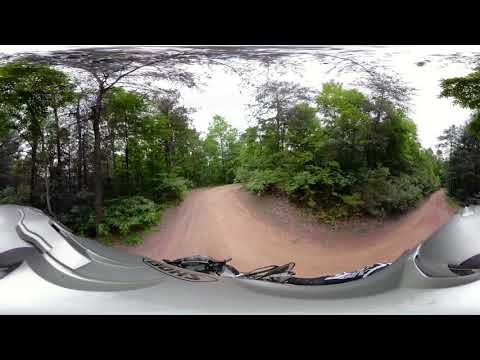This captivating image, captured from the perspective of a bike rider, offers a panoramic and somewhat fish-eyed view of a trail, evoking the sensation of moving through an expansive outdoor space. The trail itself is a blend of light brown and dark beige hues, winding its way through a lush setting dominated by green trees and shrubs, interspersed with some leafless, stark black trees. The sky overhead is a muted, cloudy gray, with hints of a very light blue, casting a subdued light over the entire scene.

The image is highly distorted in an almost surreal manner, giving an exaggerated, elongated view of the rider’s sleeves, which are black. There is a noticeable gray and silver element at the bottom, possibly part of the rider's helmet or the front of the bike, adding to the sense of motion. The distortion extends to the path, making it appear as though it curves and stretches unnaturally, enhancing the dynamic and immersive feel of the scene. This unique perspective, with its rich array of colors and intricate details, vividly captures the essence of biking through a rugged, natural trail.